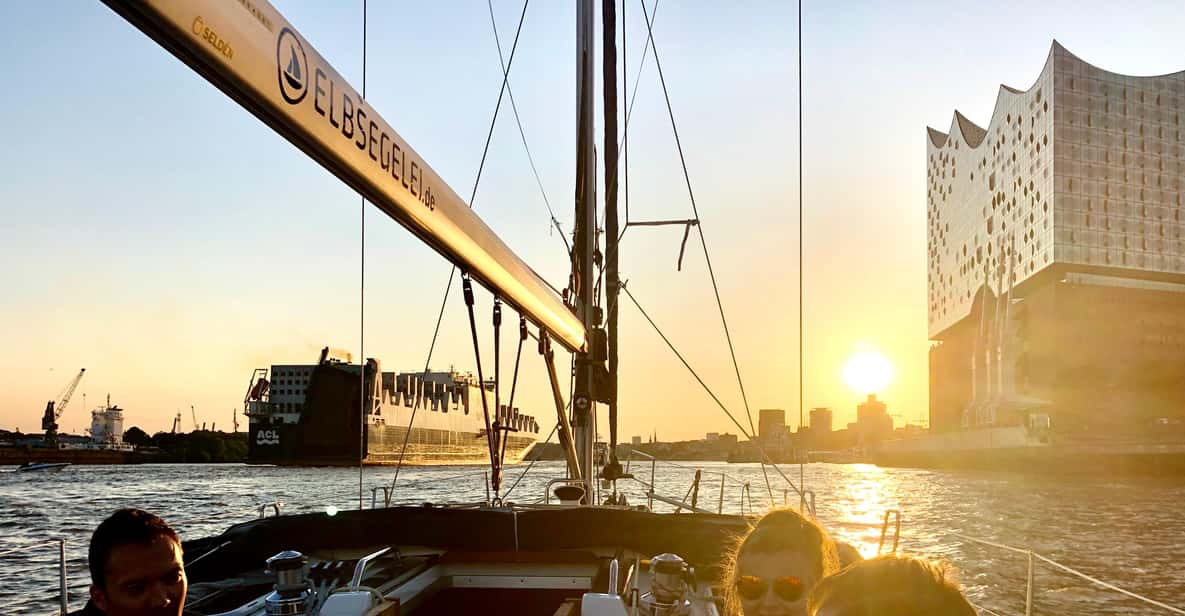The photograph captures a serene, end-of-day scene of a sailboat gliding through a large body of water, likely a river or lake, near a bustling port city. The lower half of the image prominently features the aft portion of the sailboat, which is moving away from the shore with its sail down. Seated on the benches are three individuals: a man on the left, facing the camera; and on the right, a woman wearing sunglasses with a man beside her, the woman facing the camera and the man turned towards the man on the left. They appear to be enjoying a lively conversation. The backdrop reveals a picturesque setting with the sun dipping low in the sky, casting a warm glow over the water, which looks gray in the fading light. To the right, a tall glass building stands elegantly, while the left side shows a large docked ship and a crane, hinting at the proximity to a bustling urban port. The overall ambiance conveys a mix of leisure and urban activity against the backdrop of a stunning sunset.